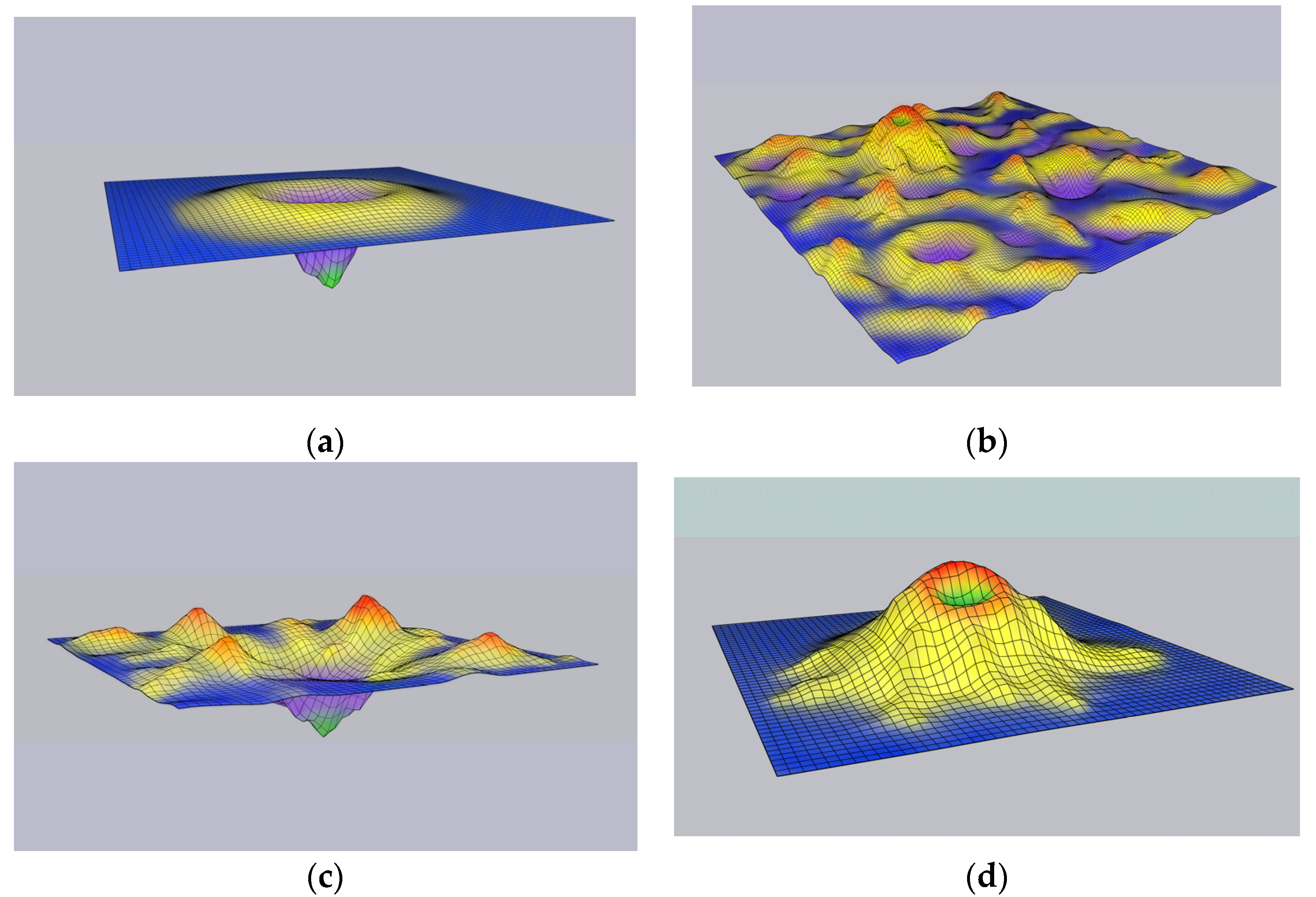The composite image consists of four 3D-rendered topographical models, each labeled A, B, C, or D, arranged in a two-by-two grid. These models depict various land formations, presumably volcanoes, characterized by their color-coded elevation contours, ranging from blue at ground level, through yellow and orange at higher altitudes, and culminating in green at the peaks.

- **Model A (Top Left)**: This depicts an inverted volcano, featuring a shallow basin atop the ocean, with a pit resembling a deep crater extending far below. The side view highlights the grid-like pattern outlining the topographic contours.

- **Model B (Top Right)**: Representing a mountainous landscape, this model showcases multiple peaks, some with visible craters. Notably, there is a large, detailed volcano with a prominent purple center amidst other smaller formations.

- **Model C (Bottom Left)**: Similar to Model A, this depicts several mountain-like structures emerging from the ocean, encircling a significant crater that plunges beneath the water, forming a distinct cavity.

- **Model D (Bottom Right)**: This features a traditional volcanic cone structure, prominently rising from the ocean, distinguished by a small crater at its summit.

Overall, these detailed 3D renderings, utilizing color gradients to illustrate elevation, provide a scientific representation of various volcanic formations.